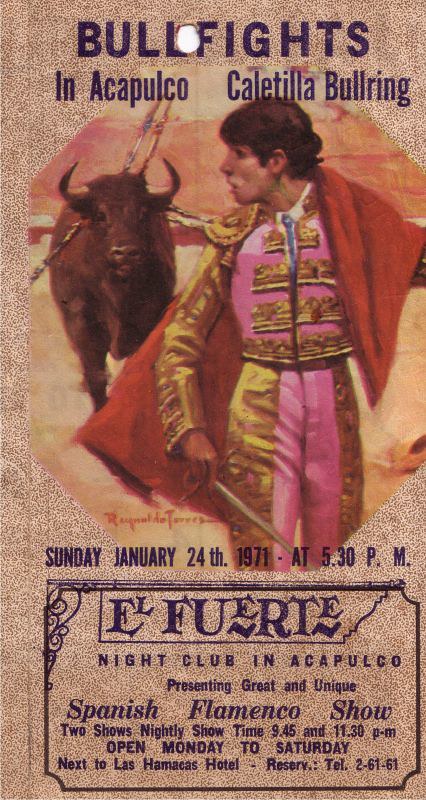This vintage advertisement from the 1970s features a tan and white stippled pattern background with bold blue lettering at the top, announcing "Bullfights in Acapulco, Calathea Bullring." It highlights a colorful and artistic photograph of a bullfighter donned in a pink outfit trimmed with gold and wielding a traditional red bullfighting sash. A brown bull is poised over his left shoulder, adding to the dramatic effect. Below this vibrant image, blue text reads: "Sunday, January 24, 1971, at 5:30 p.m. El Fuerte Nightclub in Acapulco presents a great and unique Spanish flamenco show. Two shows nightly, showtimes at 9:45 p.m. and 11:30 p.m. Open Monday to Saturday next to Las Hamacas Hotel." The ad also suggests reservations can be made via telephone number 261-61. The overall design confirms its vintage 1971 origin, emphasizing the rich cultural heritage and entertainment scene in Acapulco.